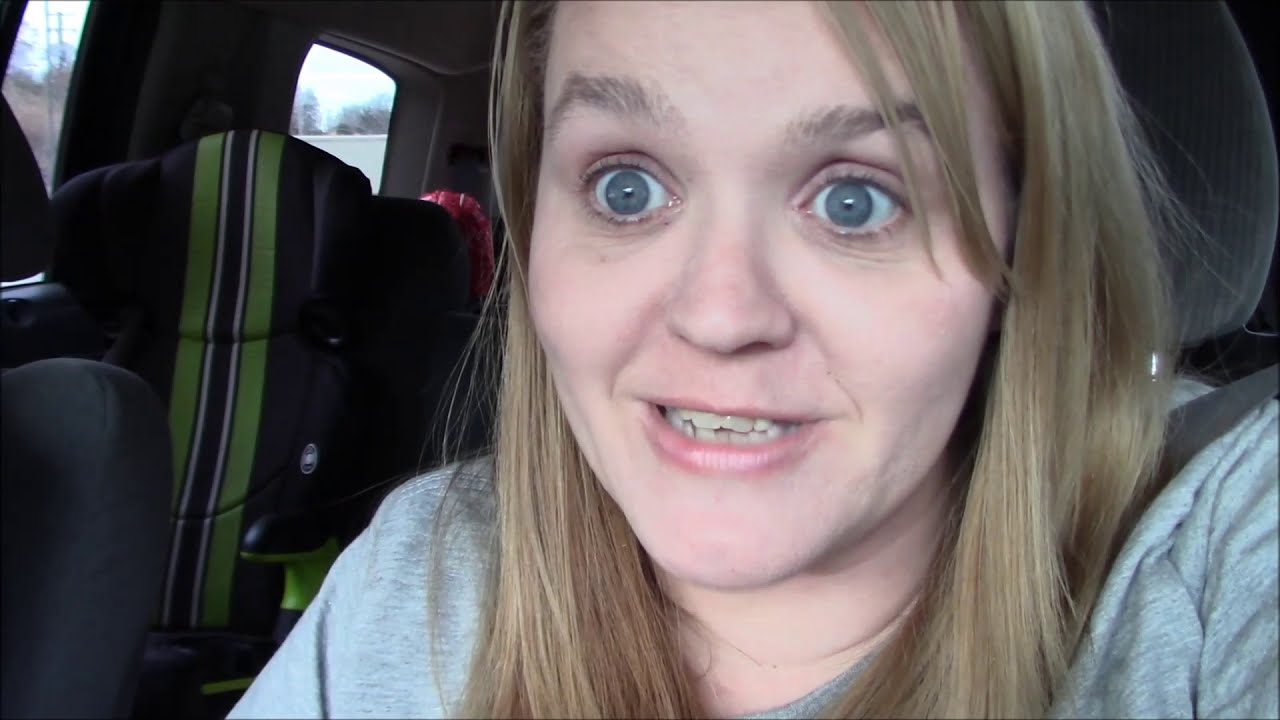In this captivating close-up photograph, a young woman with striking blue eyes and blond hair, which falls just past her shoulders, sits in the front seat of a vehicle. Her wide-eyed expression, with furrowed and raised eyebrows, conveys a sense of wonderment or surprise as she gazes slightly to the left of the camera. Her mouth is open, perhaps mid-sentence or mid-smile, revealing slightly crooked teeth. She is dressed in a gray hoodie over a gray t-shirt and is secured by a gray seatbelt.

The interior of the vehicle features dark seats with a green stripe running down one adjacent to her. Behind her, a child's car seat is visible, suggesting the presence of a baby. Out the windows, the ambient environment reveals a natural setting with trees, possibly on an overcast day, and distant telephone poles. Overall, the image draws the viewer in, largely due to the woman's expressive and mesmerizing blue eyes.